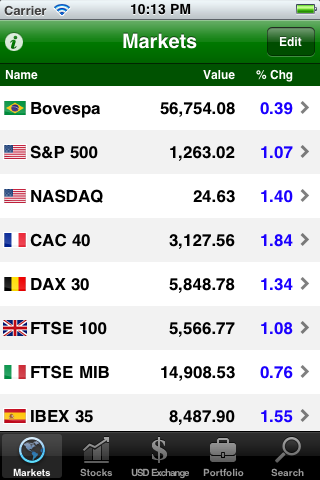This image captures a screenshot of a cell phone screen. In the upper left-hand corner, there's the word "carrier" displayed in black text. Adjacent to the right is a Wi-Fi signal icon, followed by the time, which reads 10:13 PM. Further to the right is a full battery icon, indicating the device is fully charged. 

Below this status bar is a green banner with the word "Markets" prominently displayed in white text. On the right side of this banner is an "Edit" button. 

The main display features a table divided into three columns labeled "Name," "Value," and "Percentage Change," showcasing various market indices. 

1. **BOVESPA**: 
   - **Value**: 56,754.08
   - **Change**: 0.39%

2. **S&P 500**: 
   - **Value**: 1,263.02
   - **Change**: 1.07%

3. **NASDAQ**: 
   - **Value**: 24.63
   - **Change**: 1.40%

4. **CAC 40**: 
   - **Value**: 3,127.56
   - **Change**: 1.84%

5. **DAX 30**: 
   - **Value**: 5,848.78
   - **Change**: 1.34%

6. **FTSE 100**: 
   - **Value**: 5,566.77
   - **Change**: 1.08%

7. **FTSE MIB**: 
   - **Value**: 14,908.53
   - **Change**: 0.76%

8. **IBEX 35**: 
   - **Value**: 8,487.90
   - **Change**: 1.55%

Each market is presented with its respective current value and the percentage change, providing a comprehensive overview of market performance.